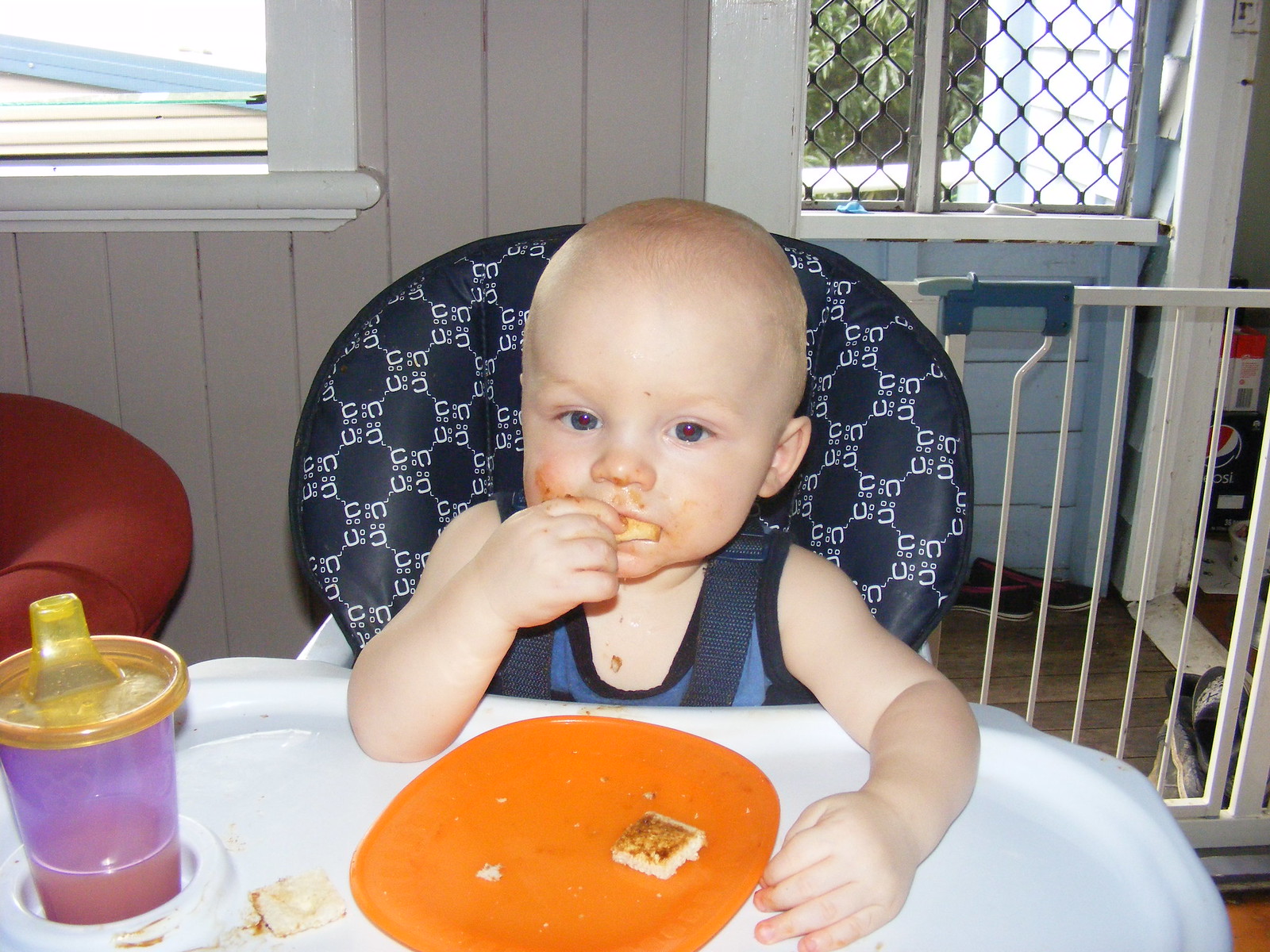In a vividly detailed photograph, there is a young toddler with piercing blue eyes, sitting in a padded high chair adorned with dark blue fabric and white rings. The child is messily eating, with food smeared across his face, while wearing a blue shirt. Strapped securely into the high chair, he engages with his meal on the white tray in front of him, which holds an orange plate filled with small squares of what seems to be toast or pancakes. The toddler uses his right hand to grasp the food, and to his left—a sippy cup with a yellow lid and purple body, containing a reddish liquid about a quarter full. The background reveals a white wooden wall with a gated window showing minimal vegetation outside. Additional homey details, like some shoes on the floor, add to the cozy domestic scene.